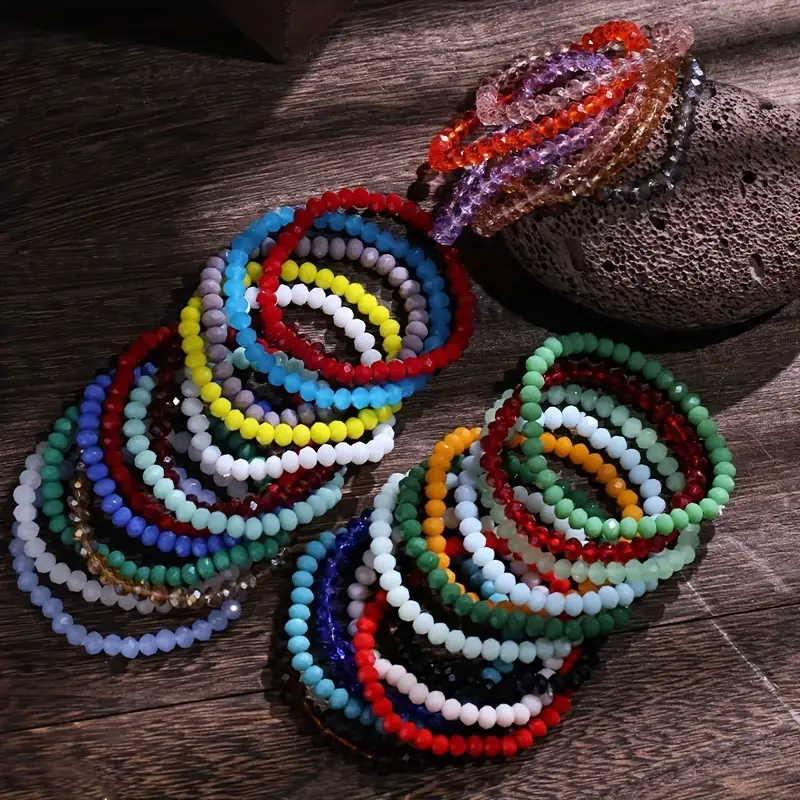This image captures a meticulously arranged display of handmade jewelry on a rustic wooden surface, set against a log wall. The focal point is two organized stacks of bracelets, each crafted from solid-colored beads, featuring vibrant hues of red, blue, yellow, white, and purple. Above these bracelets, strands of beads in more pastel and possibly clear shades suggest either larger necklaces or ongoing projects. Scattered among these items are additional strands of beads with a variety of colors such as purple, green, and white. Some of the jewelry, including both larger pearl-like stones and smaller beads, is displayed atop a flat rock on the wooden table, adding to the unique and visually pleasing presentation. This detailed assortment highlights the craftsmanship and creativity put into making these colorful and diverse pieces.